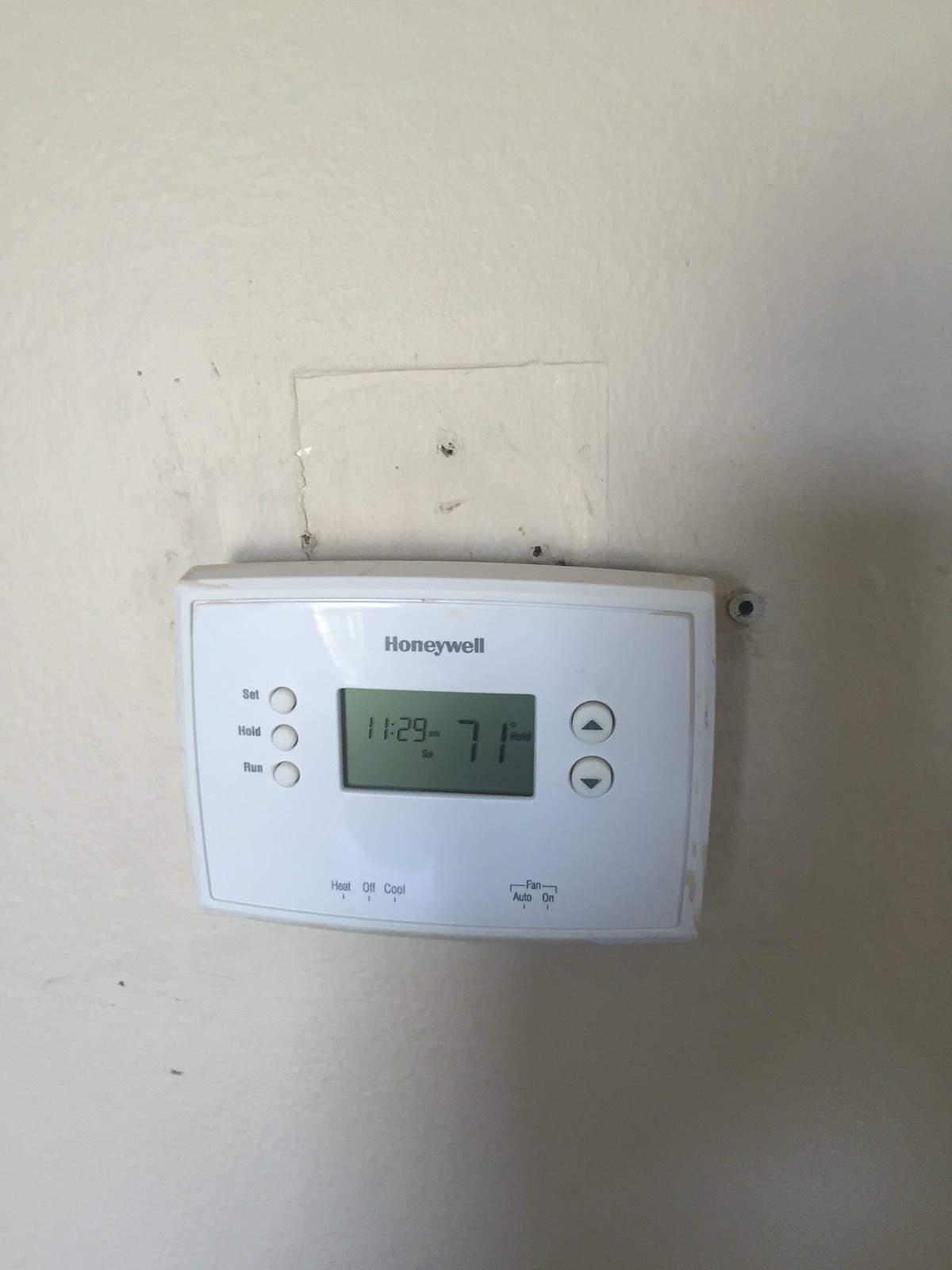The image provides a close-up view of a household thermostat mounted on a white wall. The background wall, which occupies the right center of the image and extends halfway to the left before disappearing off the bottom, casts a subtle shadow. Centrally located in the image is the rectangular thermostat, which is slightly wider than it is tall. The device's edges have a dingy white hue, while its center remains a cleaner white.

At the top center of the thermostat, "Honeywell" is displayed in black lettering. Directly below this branding is a small screen, indicating "11:29" on the left side and "71 degrees" on the right side. To the left of the screen, three buttons are visible, though their labels are unclear. On the right side of the screen, two buttons are marked with up and down arrows.

In the top right corner of the image, a small drilled hole is noticeable in the wall. Just above the thermostat, a faint outline suggests where an old thermostat might have been previously installed. This outline measures approximately two inches from the left and right sides and extends two inches upwards, forming a bordered rectangle. Below this outline, two holes are visible above the newly installed unit.

At the bottom of the screen, just beneath the "11:29" display, are three small sections, although their details are indiscernible. To the right of the thermostat, the words "Auto" and "On" can be seen.